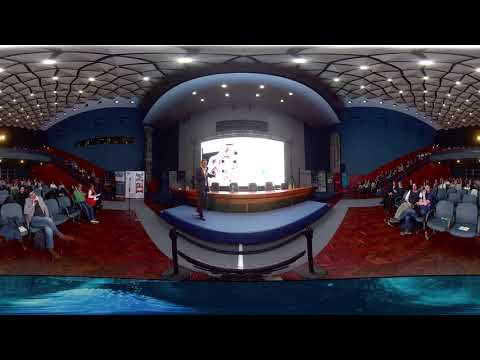The panoramic image captures a theater-like setting with a wraparound view. Central to the scene is a small blue stage positioned directly in the middle, featuring a man in a blue suit giving a performance or presentation. He is pointing towards a screen on the wall behind him, though the screen's content isn't visible. The stage is bordered by a gray trim and surrounded by red carpeting and blue walls. The high, domed ceiling above is gray with embedded lights and black stripes, contributing to a spacious and well-lit atmosphere. Rows of padded seating are arranged on both sides of the stage, populated by an audience that is not fully filling the seats, with some people standing off to the side. The audience members appear to be part of a gathering, possibly indicated by some wearing name tags. The theater's ceiling features a textured, soundproof design, adding to the acoustic quality of the environment. The photo is rich in colors, predominantly showcasing shades of blue, gray, red, turquoise, black, silver, white, and green, all contributing to the vivid and dynamic ambiance of the indoor setting.